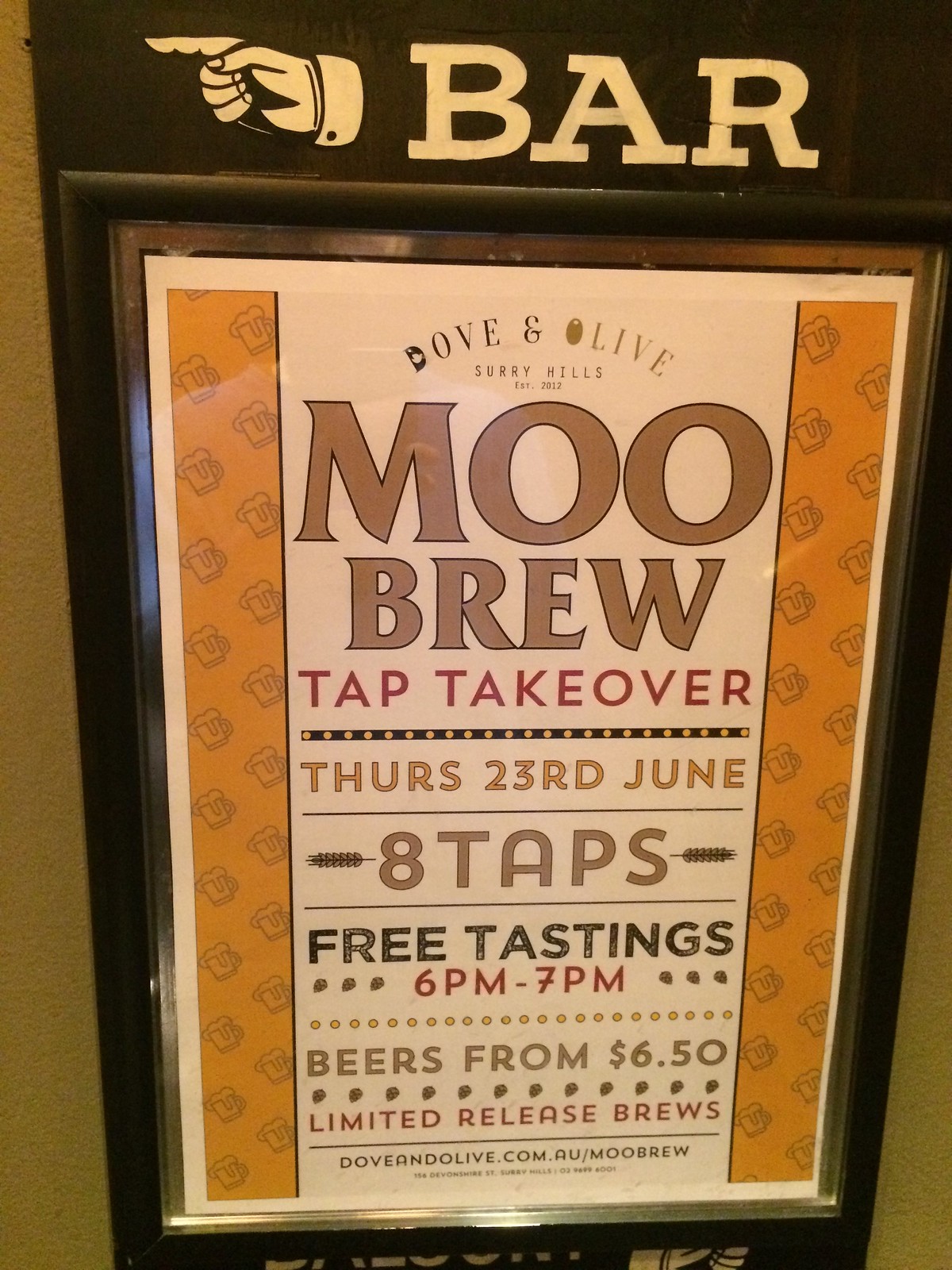This image features an advertisement for the Dove and Olive bar in Surry Hills, promoting an event called the "Moo Brew Tap Takeover." The sign, encased in a black frame and bordered by gold bars adorned with illustrations of frosty beer mugs, hangs on a brown wall. At the top of the frame, a prominent white hand points to the left with the word "BAR" in large capital letters.

The main content of the sign is set against a darker brown background. At the top, "Dove and Olive, Surry Hills, EST 2012" is prominently displayed, with the "O" in "Olive" cleverly depicted as an olive. Below, the event details are listed: "Moo Brew Tap Takeover" on Thursday, 23rd June, featuring eight taps and free tastings from 6 p.m. to 7 p.m. The phrase "free tastings" is written in black, while "6 p.m. to 7 p.m." is highlighted in red. A line of orange-yellow dots separates this section from the next, which reads "beers from $6.50" in brown print. "Limited release brews" is emphasized in red, followed by the website "doveandolive.com.au/moobrew" for more information.

At the very bottom of the sign, the address "156 Devonshire Street, Surry Hills," along with the contact number "0296996001," is listed, completing the detailed and inviting advertisement.